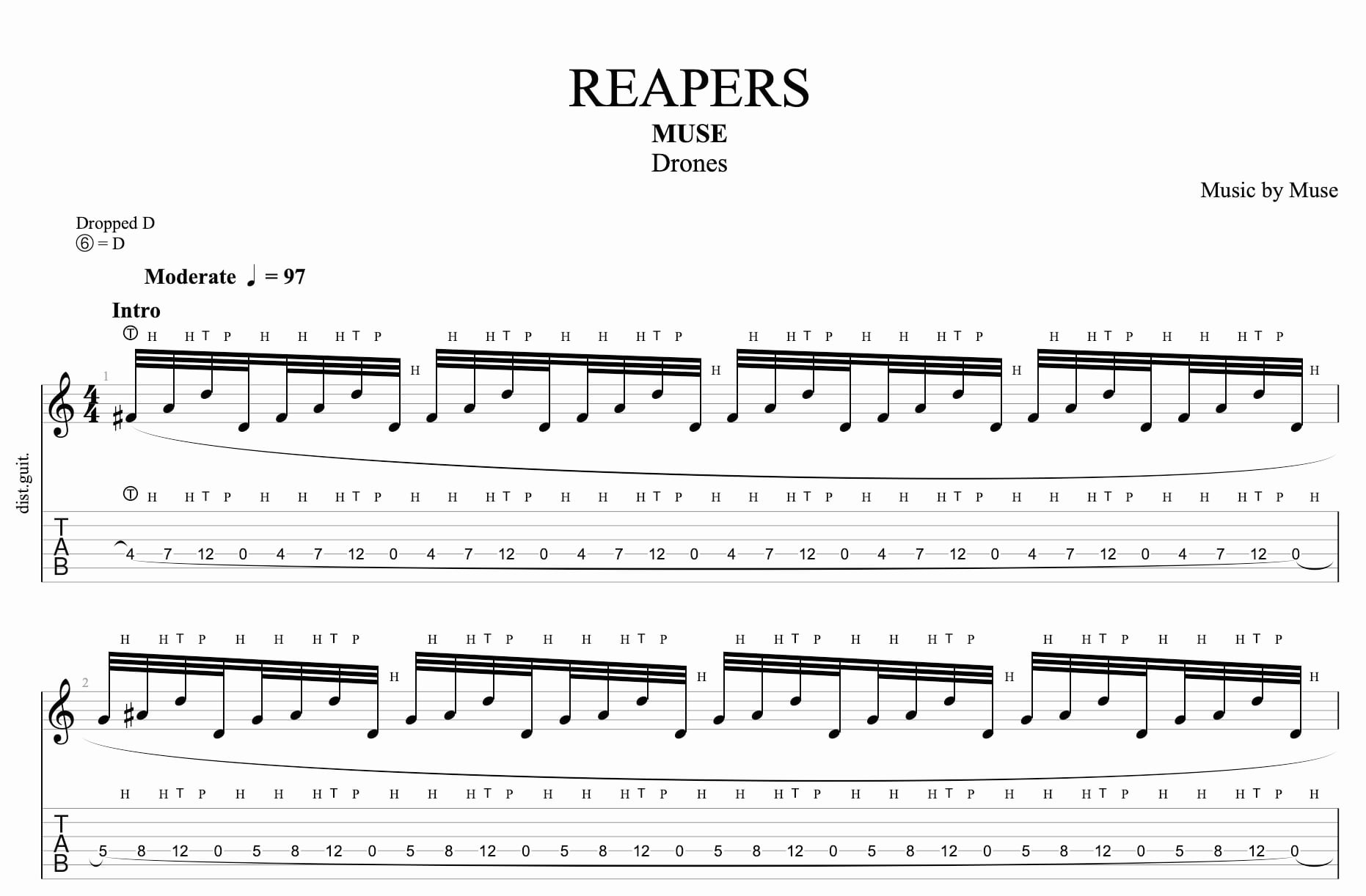The image depicts a piece of sheet music for the song "Reapers" by Muse. At the top center, the title "REAPERS" is prominently displayed in large black letters, with "MUSE" and "DRONES" written underneath it in smaller print. On the upper right corner, it states "MUSIC BY MUSE." The upper left corner notes the tuning "Dropped D," with the instructions "6 = D" and "Moderate = 97." The sheet music features two lines of musical notes, followed by guitar tabs with numbers along the horizontal lines. The main focus is on how to play the song, including the melody and guitar tabs, providing a detailed guide for playing "Reapers" by Muse.